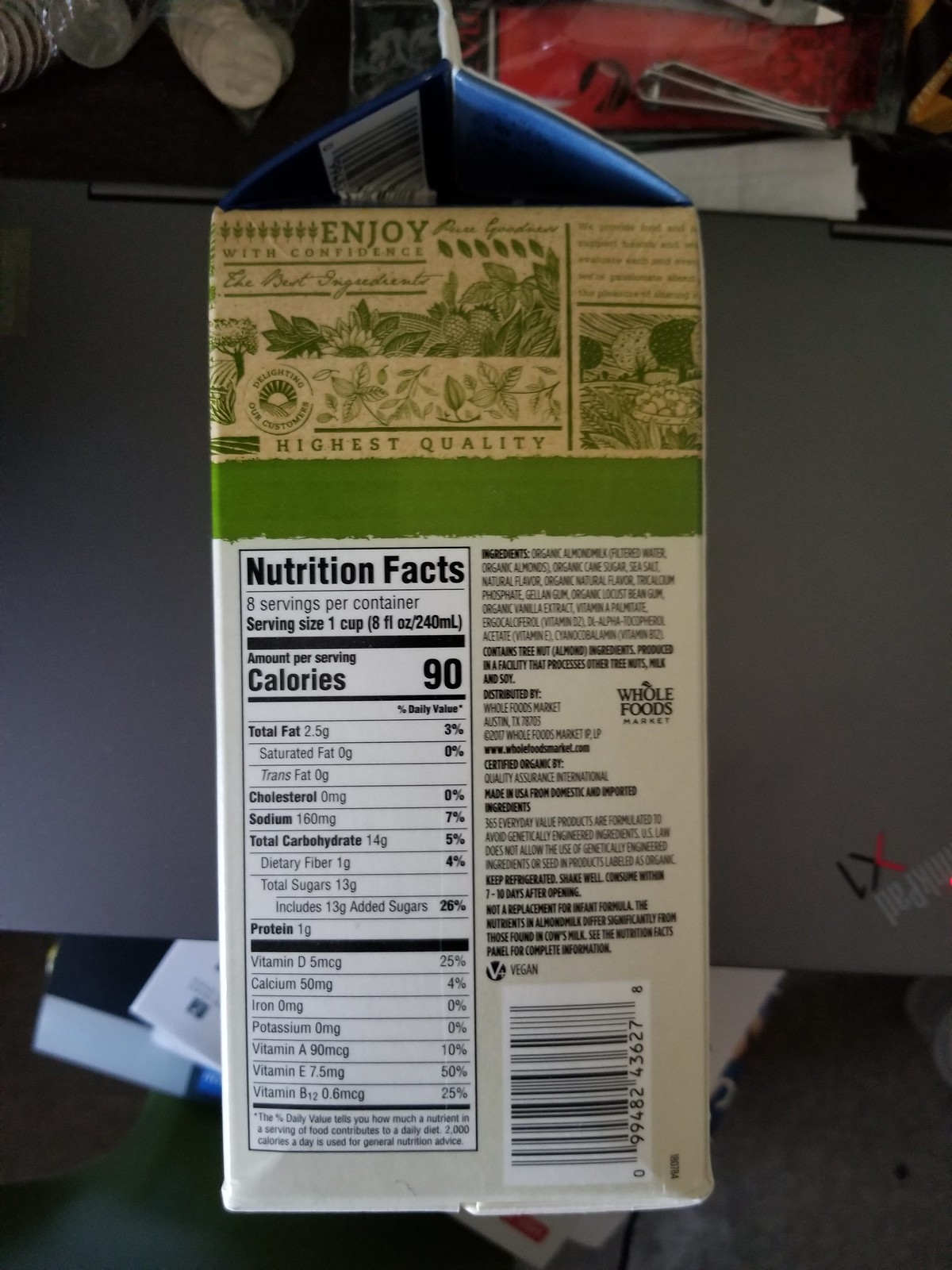This photo captures a carton of liquid, likely almond milk, lying on its side atop a surface that appears to be either a gray or silver laptop or a table. The scene extends to reveal a graystone floor beneath the table, accompanied by a few scattered items. The image focuses on the side of the carton, prominently displaying the nutrition facts and ingredients panels. The nutritional details indicate the following per serving (1 cup): 90 calories, 2.5 grams of total fat, 160 milligrams of sodium, 14 grams of total carbohydrates, 1 gram of dietary fiber, 13 grams of total sugars, and 1 gram of protein. The ingredient list starts with organic almonds, filtered water, and cane sugar, among other partially obscured elements. This photograph offers a clear view of the carton’s key nutritional information against a contrasting background.